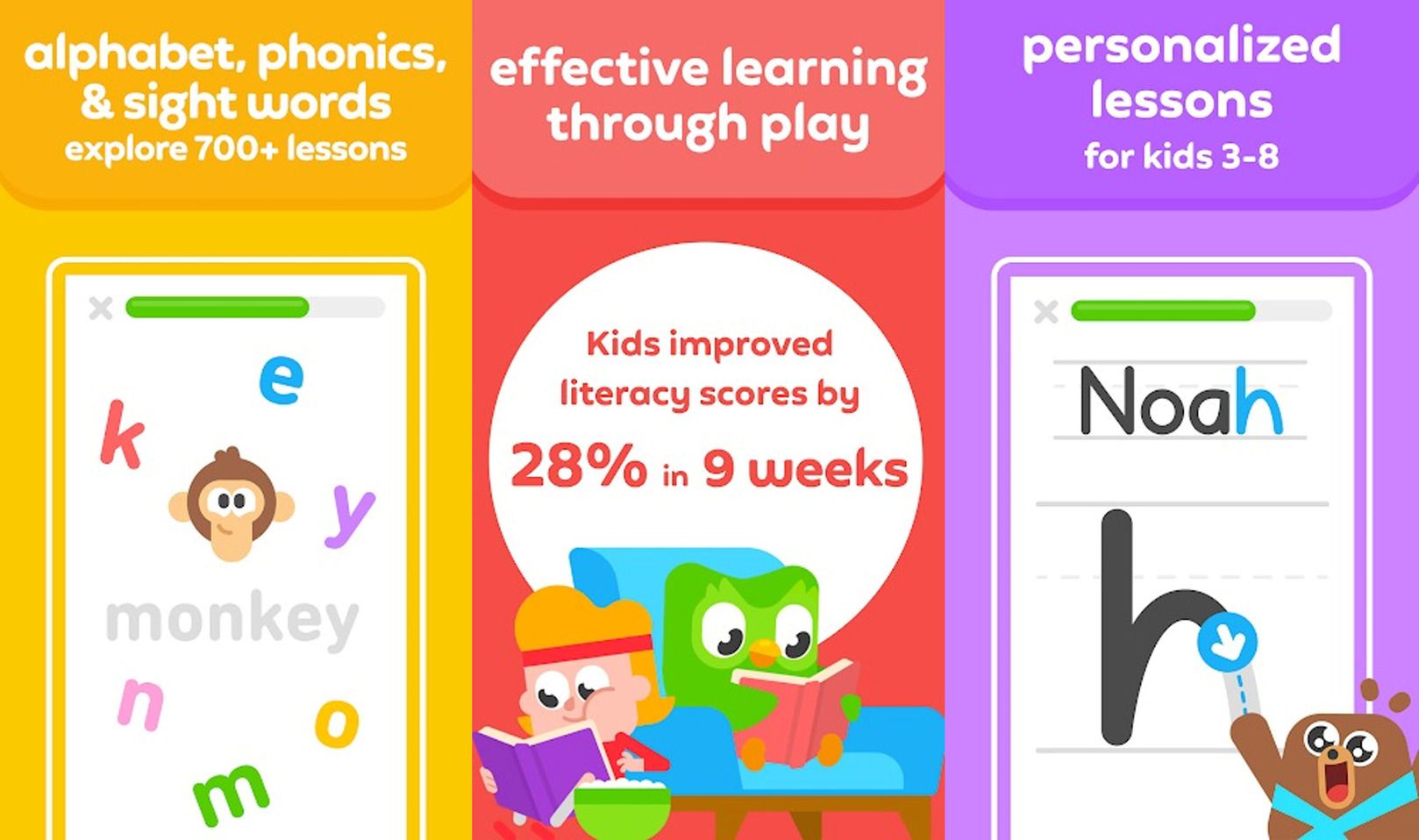This vibrant advertisement for children's educational products is divided into three equal sections with distinct colorful backgrounds. 

**Left Section:** Featuring an orange background, this section promotes "Alphabet, Phonics, and Sight Words — Explore 700+ lessons." Beneath this, an engaging image depicts a playful monkey surrounded by the letters spelling "MONKEY." Each letter is painted in a different vibrant color: red 'K', blue 'E', purple 'Y', pink 'N', green 'M', and yellow 'O'. 

**Middle Section:** Set against a red background, this part emphasizes "Effective Learning Through Play." In a large white circle with bold red text, it states, "Kids Improve Literacy Scores by 28% in 9 Weeks." Below, an adorable scene shows a green owl with glasses sitting on a blue chair, engrossed in reading a red hardcover book. On the floor next to the chair, a child with a red headband is sitting, also reading a purple book, with a bowl of popcorn placed beside them, adding a cozy touch.

**Right Section:** With a purple background, this section highlights "Personalized Lessons for Kids 3 to 8." Below, an image shows a piece of paper with "Noah" written at the top — 'NOA' in black print and 'H' in blue print. At the bottom of the screen, a charming creature, possibly a bear, traces the letter 'H' on the page, illustrating the interactive and personalized nature of the lessons. 

This detailed visual breakdown captures the essence of the learning products geared towards enhancing children's literacy through fun and engaging methods.